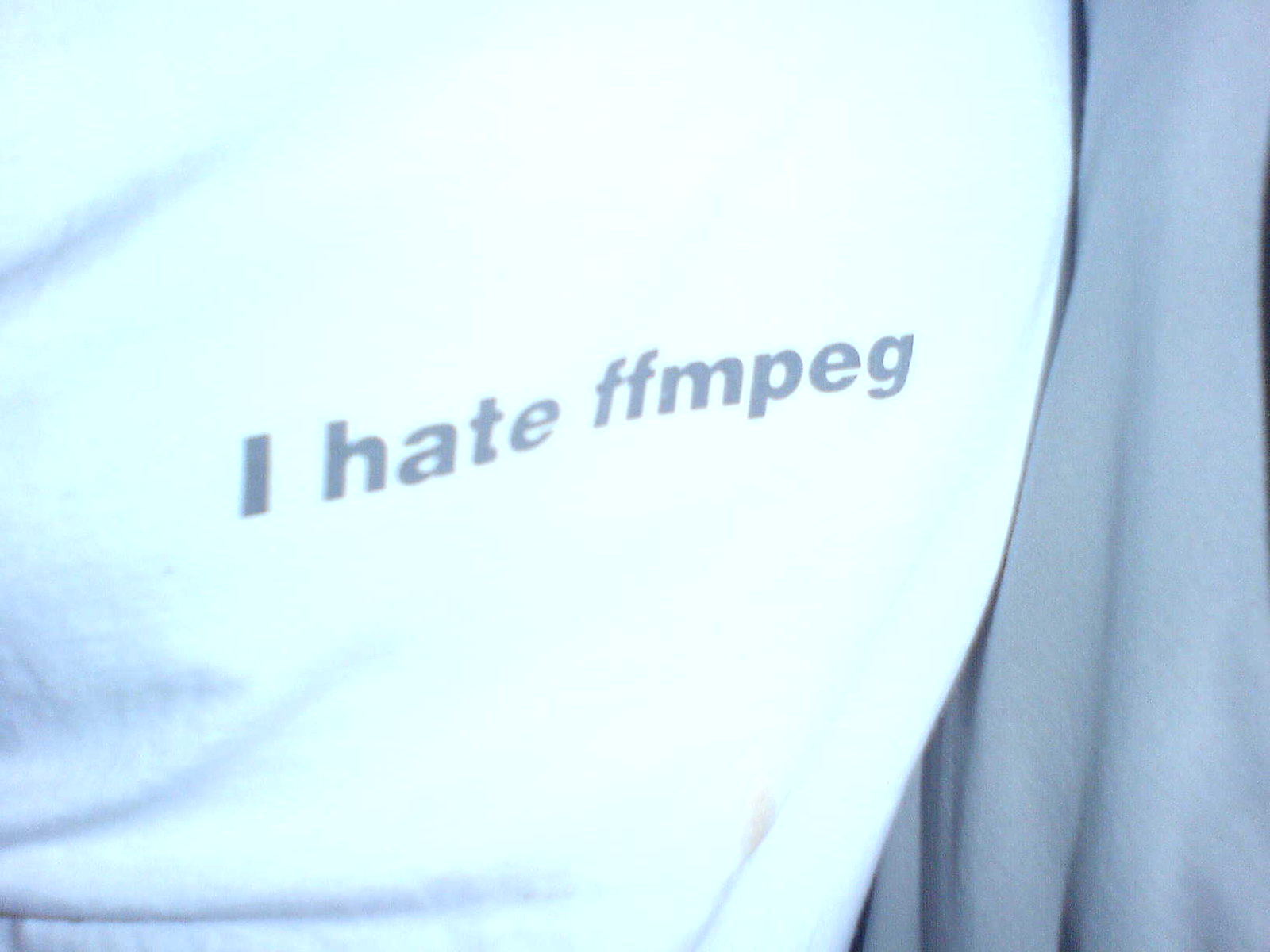A close-up shot reveals textured fabric draped over an indiscernible body part. The main fabric, a stark white material, prominently displays the handwritten words "I hate F F M P E G" in a slightly irregular font. To the right, another fabric, this one in a delicate pale gray hue, cascades vertically, adding a contrasting yet harmonious layer to the composition. The monochromatic palette of the image, limited to shades of white and gray, accentuates the textures and handwritten message, creating a nuanced and thought-provoking visual.